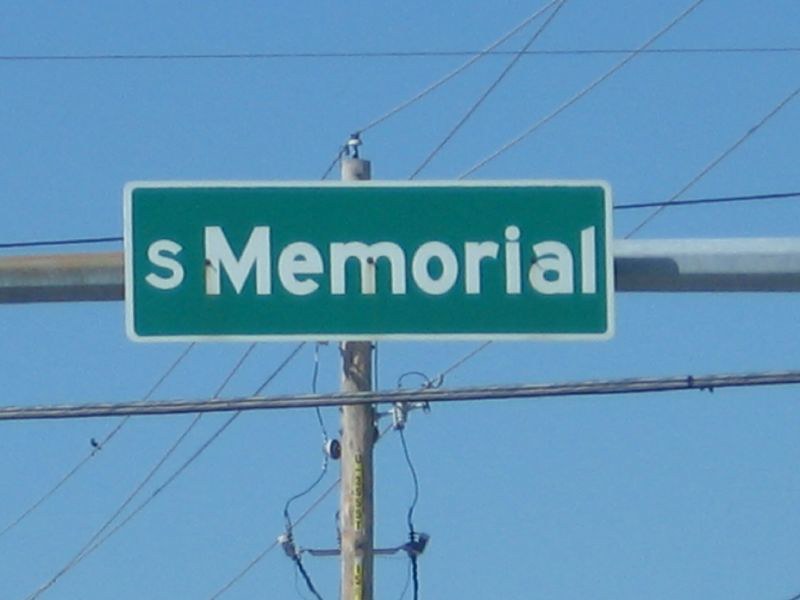In this photograph, a green rectangular street sign marked "S Memorial" with bold white letters and a white border stands out prominently. The sign is affixed to a beige telephone pole, which is partly visible and features some yellow and black writing near its base. Spread out from the pole are multiple telephone wires, crisscrossing in various shades of gray, running both diagonally and horizontally across the image. High above, set against a bright, clear, medium blue sky devoid of clouds, a small bird perches delicately on one of the wires to the left. This close-up captures only the upper portion of the pole and wires, emphasizing the sign against the expansive blue background.